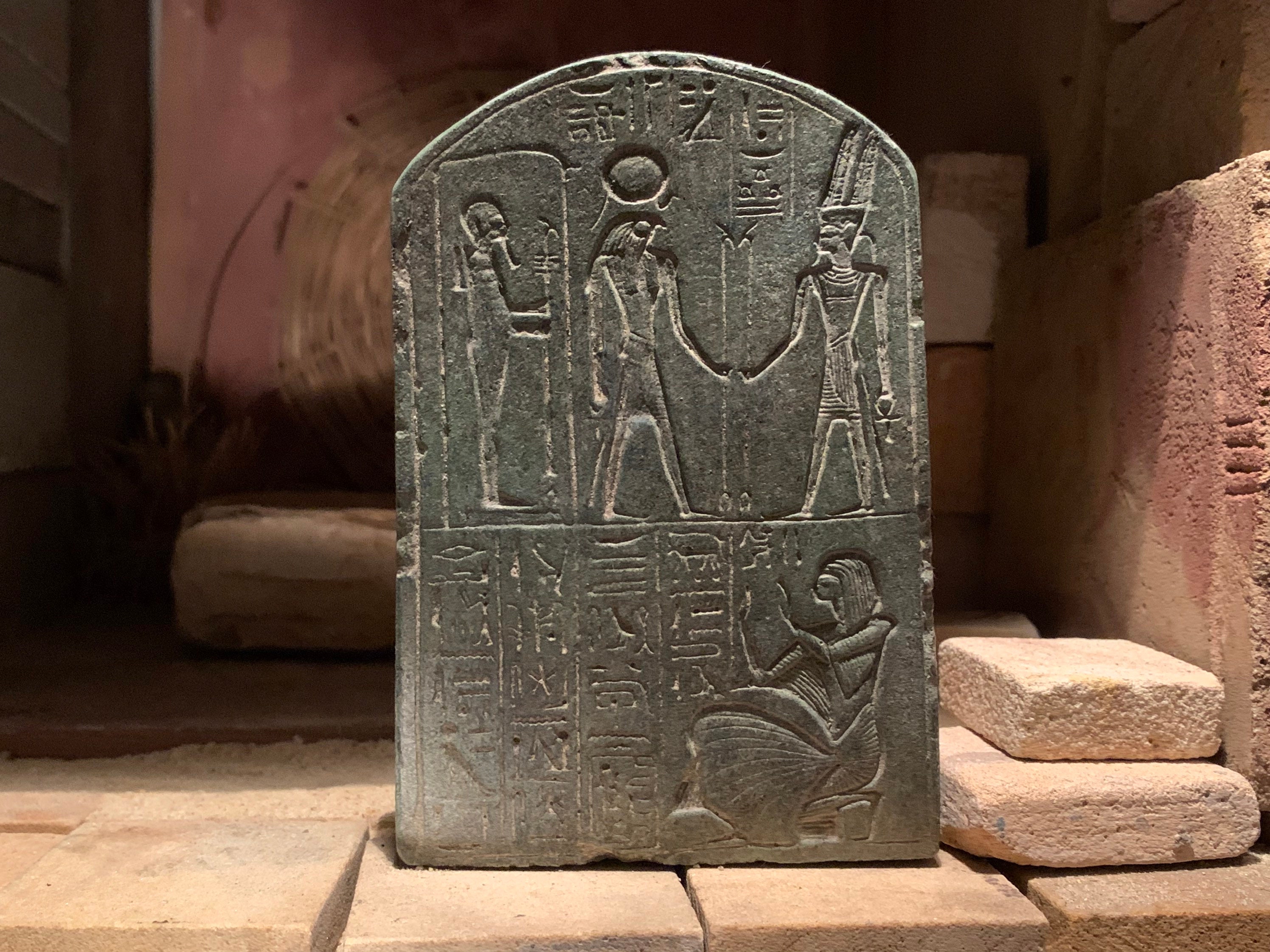In the image, a prominent stone tablet with intricate Egyptian hieroglyphs stands in the foreground, resembling a tombstone set upon a rock. The tablet appears metallic, possibly solid silver, but also retains a stone-like gray appearance. This detailed artifact is adorned with ancient carvings: on the far left, an older man, perhaps a priest or noble, holds a staff; in the middle, the sun god Ra, identifiable by the sun depicted above his head, appears to be interacting with another figure presumed to be a goddess, possibly Nefertiti, distinguished by her elegant tall headpiece. Below, there is a depiction of a kneeling individual looking towards other hieroglyphs. The scene features heads of animals facing each other, adding to the artifact's mystique. The background is filled with reddish-tan sandstone blocks, reminiscent of an Egyptian pyramid's interior, adding depth and context to the historical significance of the tablet.